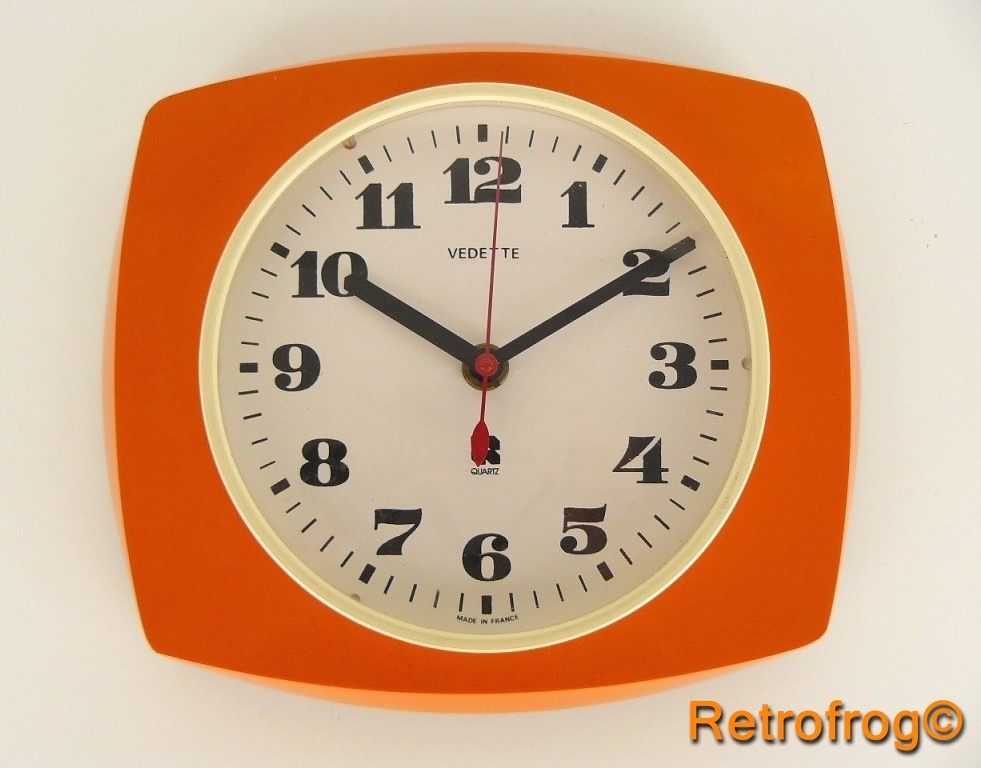The image captures a vintage alarm clock situated in the bottom right-hand corner. The clock belongs to Retro Frog Incorporated, as indicated by the orange text and circled 'C' beside it. Reflecting a 1970s aesthetic, the clock features a bold orange plastic casing, a popular color choice from that era. This French-made quartz clock, crafted by VEDETTE, showcases a classic circular face with standard numerals from 1 to 12. The current time displayed on the clock is precisely 10:10. The red second hand is almost vertically aligned at the 12 o'clock position, adding a vibrant contrast to the timepiece. Additionally, the clock's face is accentuated by a yellow-orange circle, highlighting the clock's retro design.